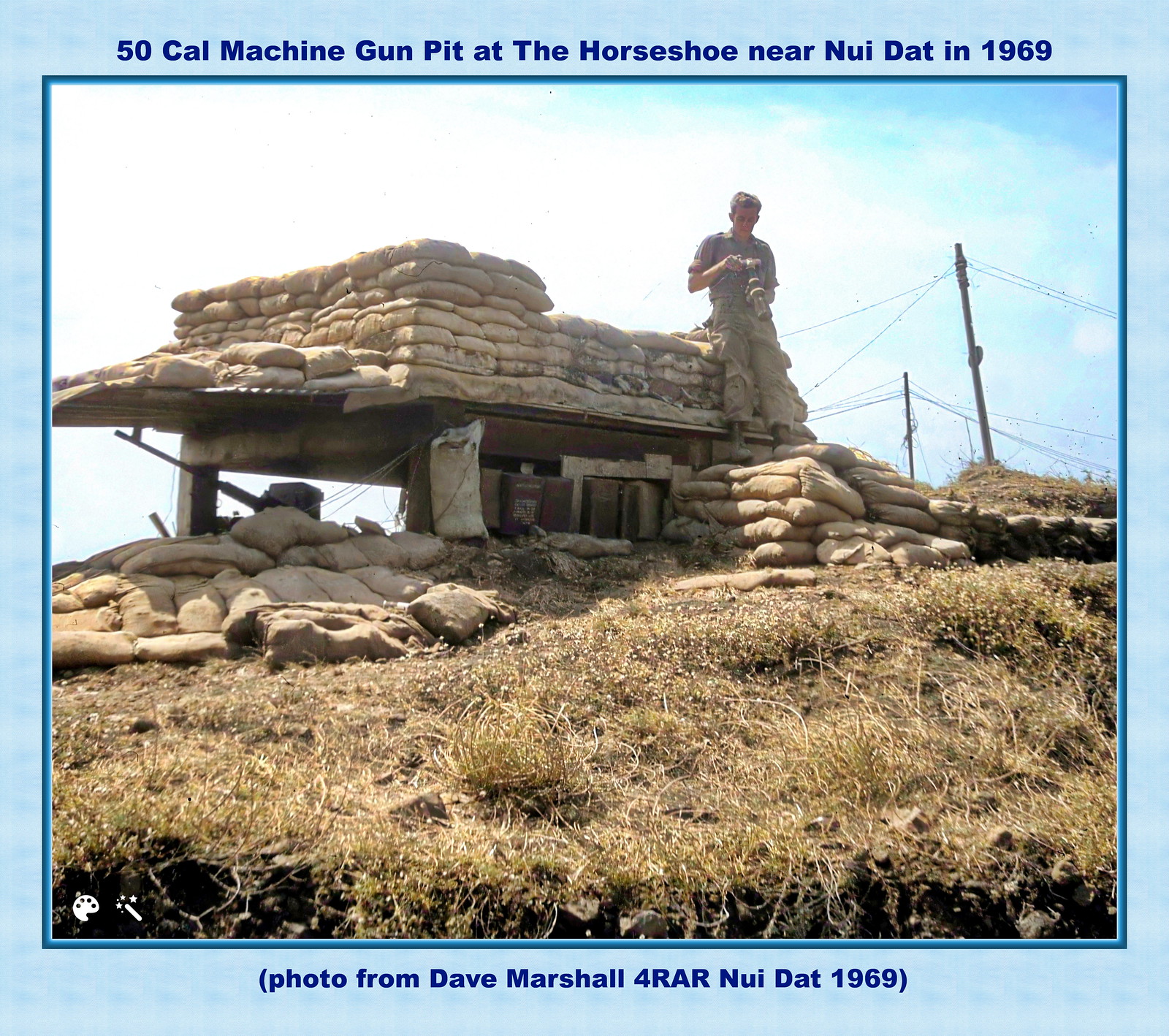This detailed full-color photograph captures a combat zone scene from 1969 in Vietnam, specifically at the "50 Cal Machine-Gun Pit at the Horseshoe near Noydat," with Noydat spelled N-U-I-D-A-T. The image is framed with a blue border that includes this descriptive title at the top, while the bottom credits the photo to Dave Marshall for 4RAR Noydat 1969. The focal point is a soldier clad in an all-beige military uniform, complete with cargo pants and boots, standing atop sandbag fortifications. The large .50 caliber machine gun is prominently featured, positioned within the trench area fortified by numerous beige sandbags. The background reveals dry, dead grass under a blue sky punctuated by clouds, and a network of power lines and telephone poles. The overall scene highlights a desolate environment indicative of a wartime setting.